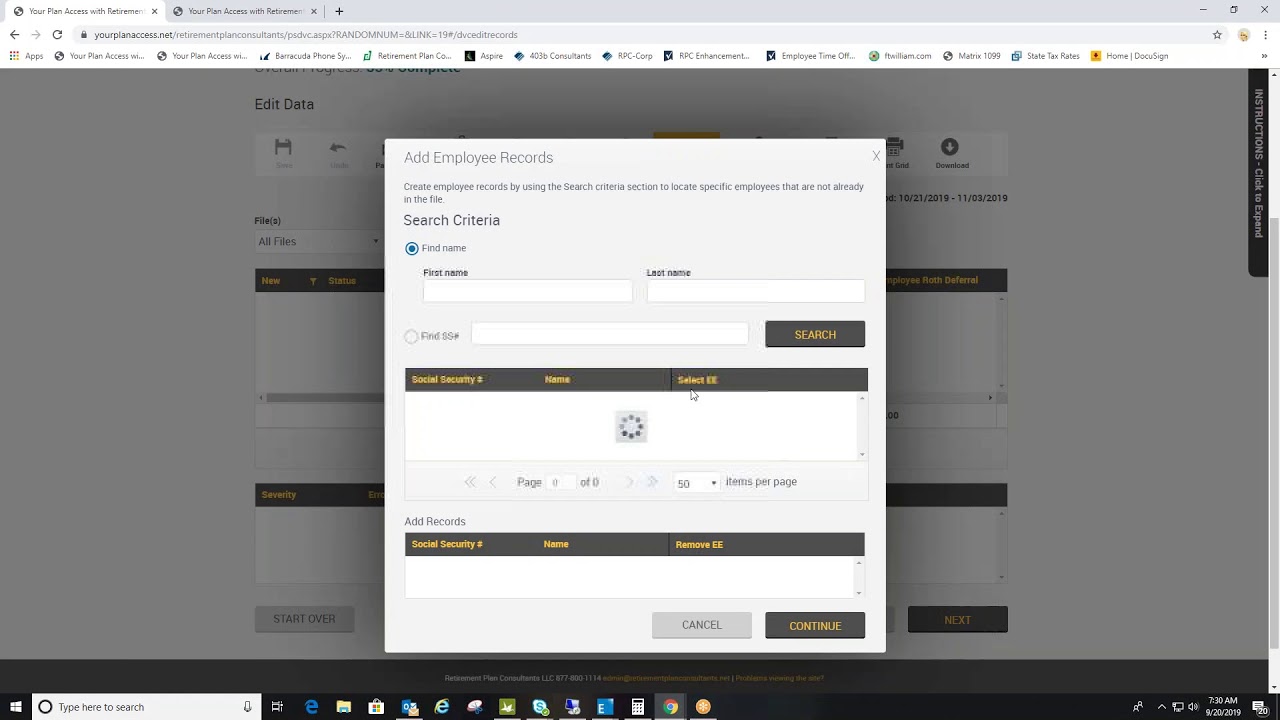The screenshot captures a web page being displayed in the Google Chrome browser on a Windows operating system. The specific URL appears to be related to a retirement plan management site, indicated as "planaccess.net/retirementplanconsultants/PS_DVC.aspx?randomNUM".

The focal point of the screenshot is a large, gray rectangular box titled "Add Employee Records". This section provides instructions for creating employee records by using the search criteria fields to locate employees who are not already in the system.

The gray box contains the following elements:
1. **Search Criteria Section**:
   - **Find Name**: This includes fields to input the first name and last name of the employee. The first name field has a blank white box where data can be entered, and the last name field is similar.
   - **Find SS Number**: Below the name fields, there is a field labeled "Find SS Number" with another blank box for entering a Social Security Number.

2. **Search Results Table**:
   - A table underneath the search criteria section lists employees with columns for Social Security Number, Name, and a select option. At the time captured, the table appears to contain zero items with a pagination control indicating "Page 0 of 050 items per page". There is a loading icon, represented by a circle made up of dots.

3. **Control Buttons**:
   - Below the results table, there are two buttons: "Add Records" and "Continue". The "Add Records" button is distinctive with its black background and gold writing, featuring the labels Social Security Number, Name, and Remove.

This web interface is designed to facilitate the addition of employee records by locating existing employees through specific search criteria, and then allowing the user to add them to the records list via the provided controls and fields.